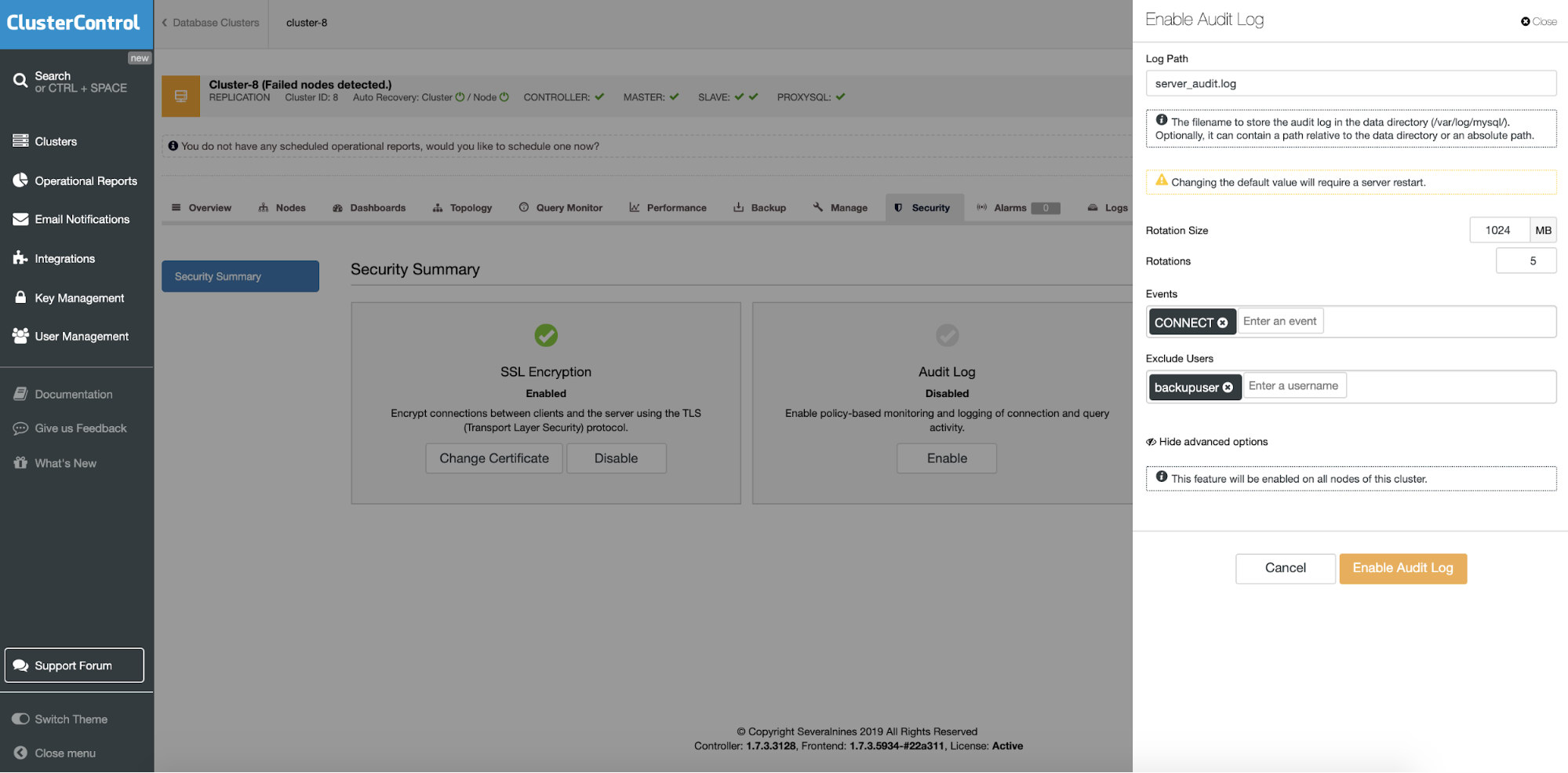This screenshot showcases a detailed view of a software dashboard. In the top left corner, a prominent blue rectangle displays the text "Cluster Control" in white. A dark grey sidebar on the left-hand side features a series of navigation buttons, each adorned with white icons and text. There are seven primary white buttons followed by three grey buttons for additional functions. The central section of the dashboard, with a slightly black-tinted grey background, contains two rows of navigational tabs. On the far right of the dashboard lies an option labeled "Enable Audit Log," neatly positioned for easy access.